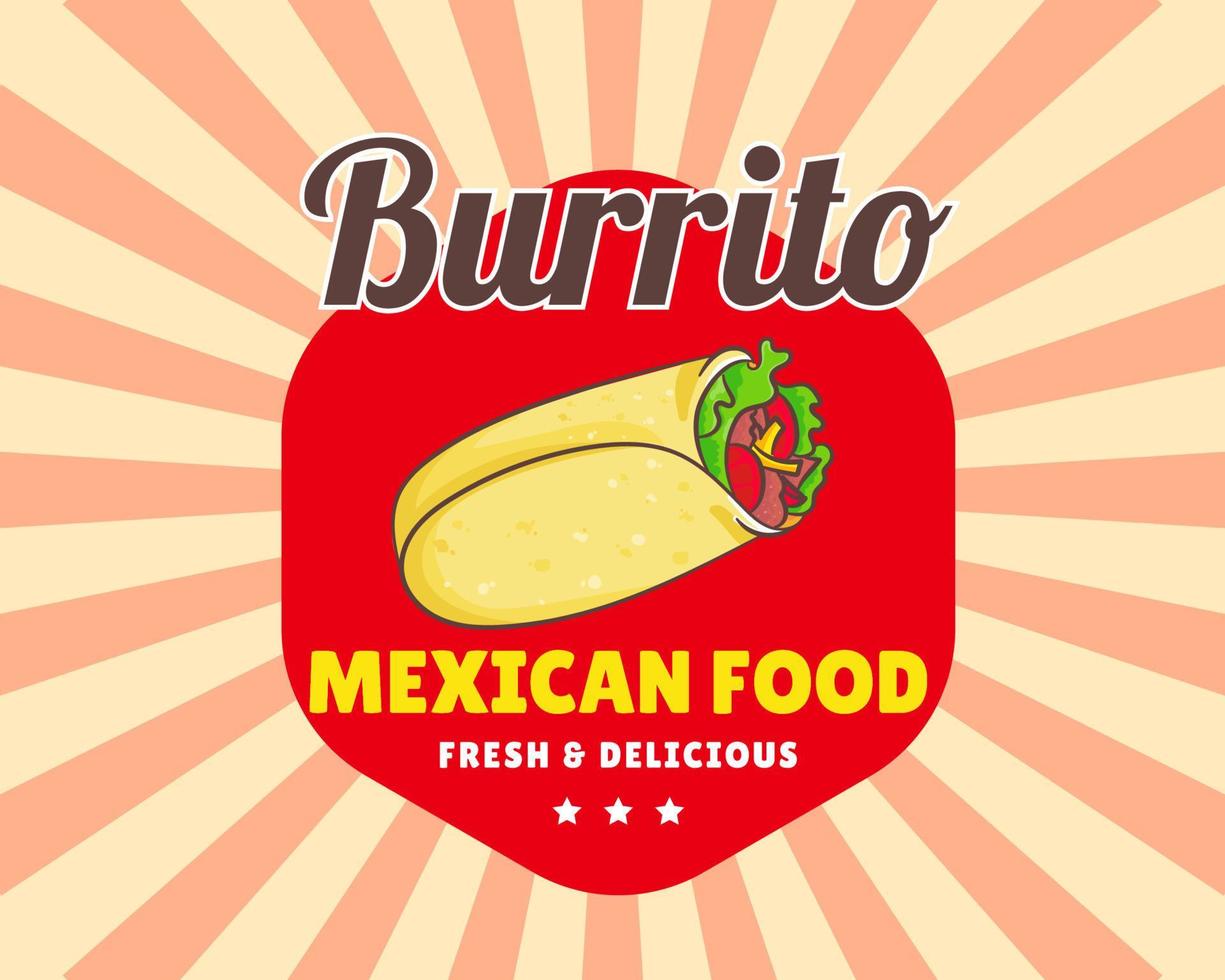The image presents an alluring advertisement for Mexican cuisine, dominated by a bold and vibrant red hexagonal logo at its center. The top of the hexagon prominently displays the word "Burrito" in large, brown lettering with a white outline. Just beneath this bold title, there is a detailed illustration of a tantalizing burrito, bursting with vibrant fillings including crisp lettuce, juicy tomatoes, savory steak, and melted cheese, depicted in rich yellows, greens, reds, and browns.

Below this mouth-watering illustration, the phrase "Mexican Food" is clearly written in bright yellow text. Beneath that, in white lettering, the enticing words "Fresh and Delicious" are displayed, accompanied by three white stars. The entire text and image composition are neatly enclosed within the red hexagonal shape.

Radiating from behind this central hexagon, a starburst pattern of alternating pale or transparent peach and beige lines extends outward, creating a dynamic backdrop that draws the eye towards the appetizing focal point. This design element enriches the overall appeal of the advertisement, emphasizing the fresh and delicious promise of the Mexican burrito.